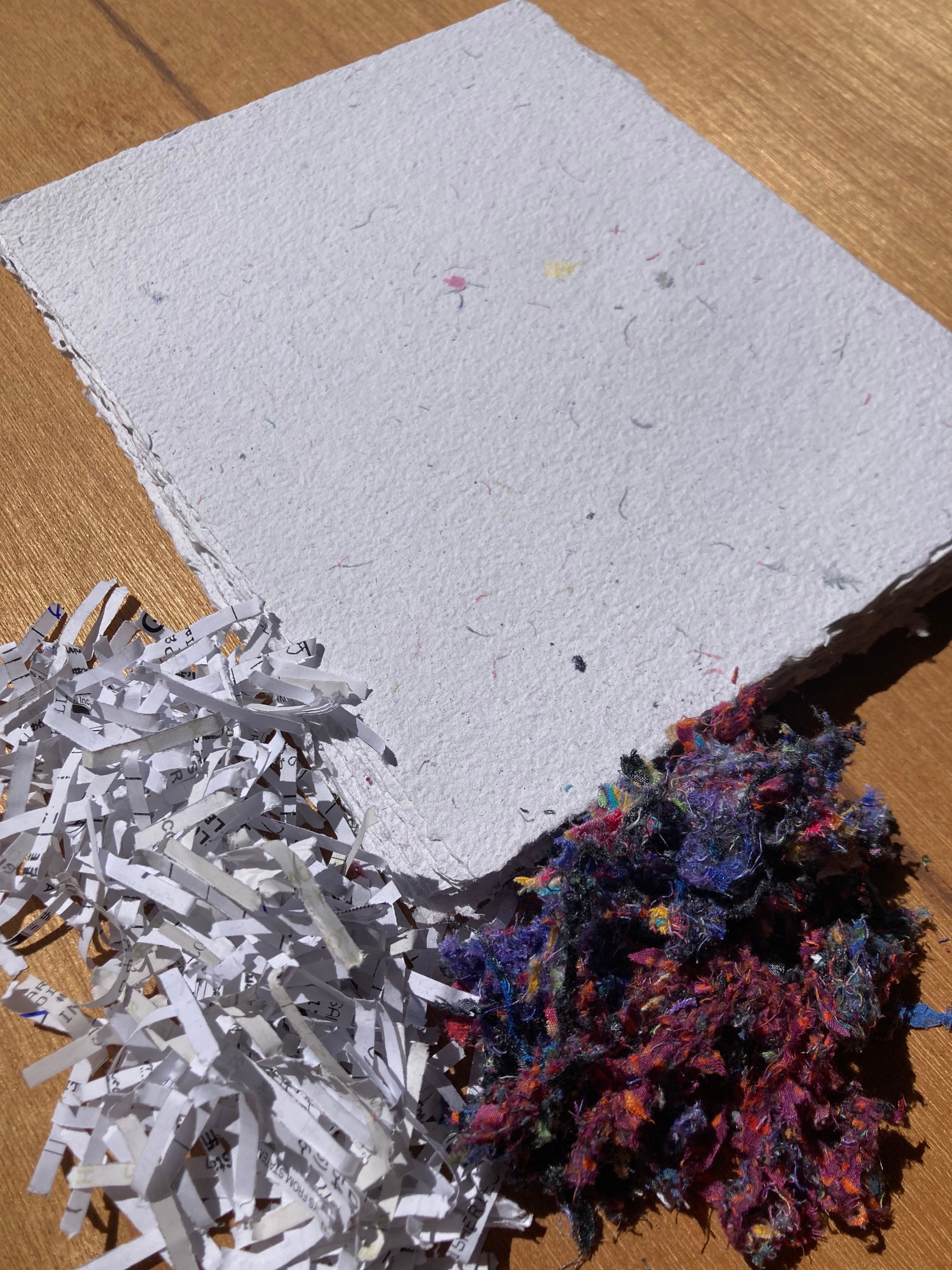In this extremely zoomed-in image, we see a light brown wooden table serving as the backdrop. Dominating the foreground is what seems to be a rough-edged, gray square that resembles a piece of drywall or a felt notebook. To the left of this square, there is a pile of shredded paper strips in light gray and white, creating a scattered, messy appearance. On the right side of the gray square, there is a mix of dark purple, blue, and pink materials that looks like a collection of lint or torn colorful felt paper. The colorful lint-like material appears layered, with a dark purple base and lighter blues and pinks interwoven at the top, adding texture to the scene.